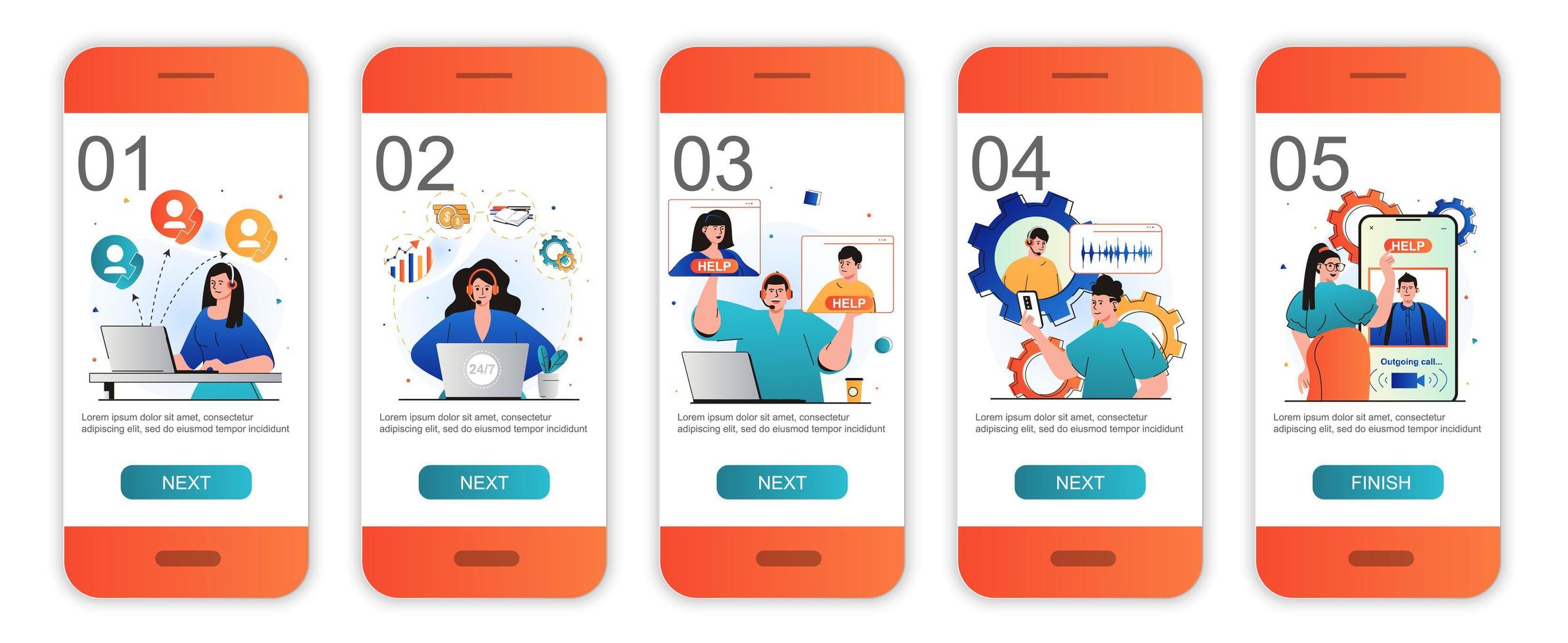The image showcases a series of five vertically-oriented panels, each representing a step in a process, likely related to customer support or a buying journey. The panels are displayed on devices resembling iPhones with distinctive orange accents at the top and bottom, and each panel is labeled numerically from 01 to 05 in the top left corner. 

**Panel 01** features an illustration of a woman in a blue shirt with a headset, typing on her laptop, likely representing a customer service agent. Accompanying this scene are colorful bubbles (blue, red, and yellow) depicting simplified human figures, and a 'Next' button in teal at the bottom.

**Panel 02** shows another woman with longer hair, also wearing a headset and engaging with her laptop. Above her, symbols are faintly visible, potentially indicating data or analytics. Like the first panel, this one is labeled '02' and includes a 'Next' button.

**Panel 03** illustrates a man in a teal shirt holding up two smaller panels of a woman in blue and a person in yellow, flanked by a laptop and a coffee cup on either side. The panel, marked '03', appears to depict a help or support interface with a recurring 'Next' button below.

**Panel 04** depicts a man in a teal shirt holding a yellow gear, with additional gears and possibly an audio frequency symbol present. This step, labeled '04', suggests a troubleshooting or technical assistance phase. 

**Panel 05** shows a woman with a ponytail and glasses, wearing a blue shirt and orange pants, interacting with a phone screen that displays a help button and the silhouette of a person in blue. Behind her are overlapping blue and orange gears. The final panel, numbered '05', concludes the sequence with a 'Finish' button.

Overall, the detailed depictions in each panel collectively illustrate a structured, multi-step process involving customer service, technical support, and user interaction, presented through consistent orange-accented interfaces.